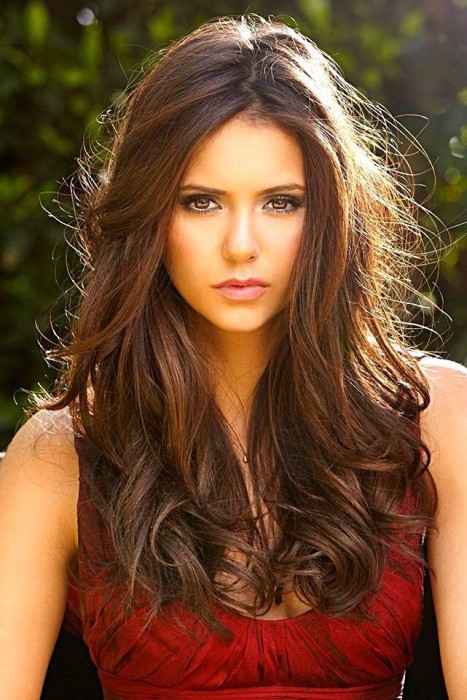The photograph features actress Nina Dobrev, captured from the waist up, exuding a youthful allure with her long, wavy hazel-brown hair cascading over her breasts. She is adorned in a sleeveless red dress that reveals a portion of her chest, complemented by subtle pink makeup and eye shadow that highlight her striking hazel eyes. Her lips are painted a soft pink. Nina's pensive expression is directed downwards, a mood emphasized by the soft sunlight that casts a gentle glow on her left shoulder and hair. The background, though blurred, suggests a serene, natural setting with green plants and trees, adding to the tranquil ambiance of the scene.